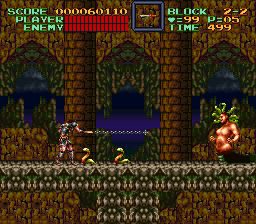A screenshot from a retro video game with classic pixelated graphics depicts an intense battle scene. The user interface in the top left corner of the screen shows three key indicators: SCORE (000060110), PLAYER, and ENEMY, with the latter two represented by red health bars. Central to the gameplay area is a gray square displaying a brown-handled silver knife, next to the text "BLOCK 2-2," "HEART = 99," "P = 05," and "TIME = 499." The character, resembling a gladiator, is minimally clothed but equipped with shoulder pads, chest armor, a skirt, and shin guards. He is in the midst of battle, throwing a chain at two green and orange snakes in front of him. On the right side of the screen, a large creature with green spiky hair, a green tail, and exaggerated features including large breasts, adds to the scene's tension. The action is set against a castle backdrop made of brown bricks with a gray-brick path running through it.